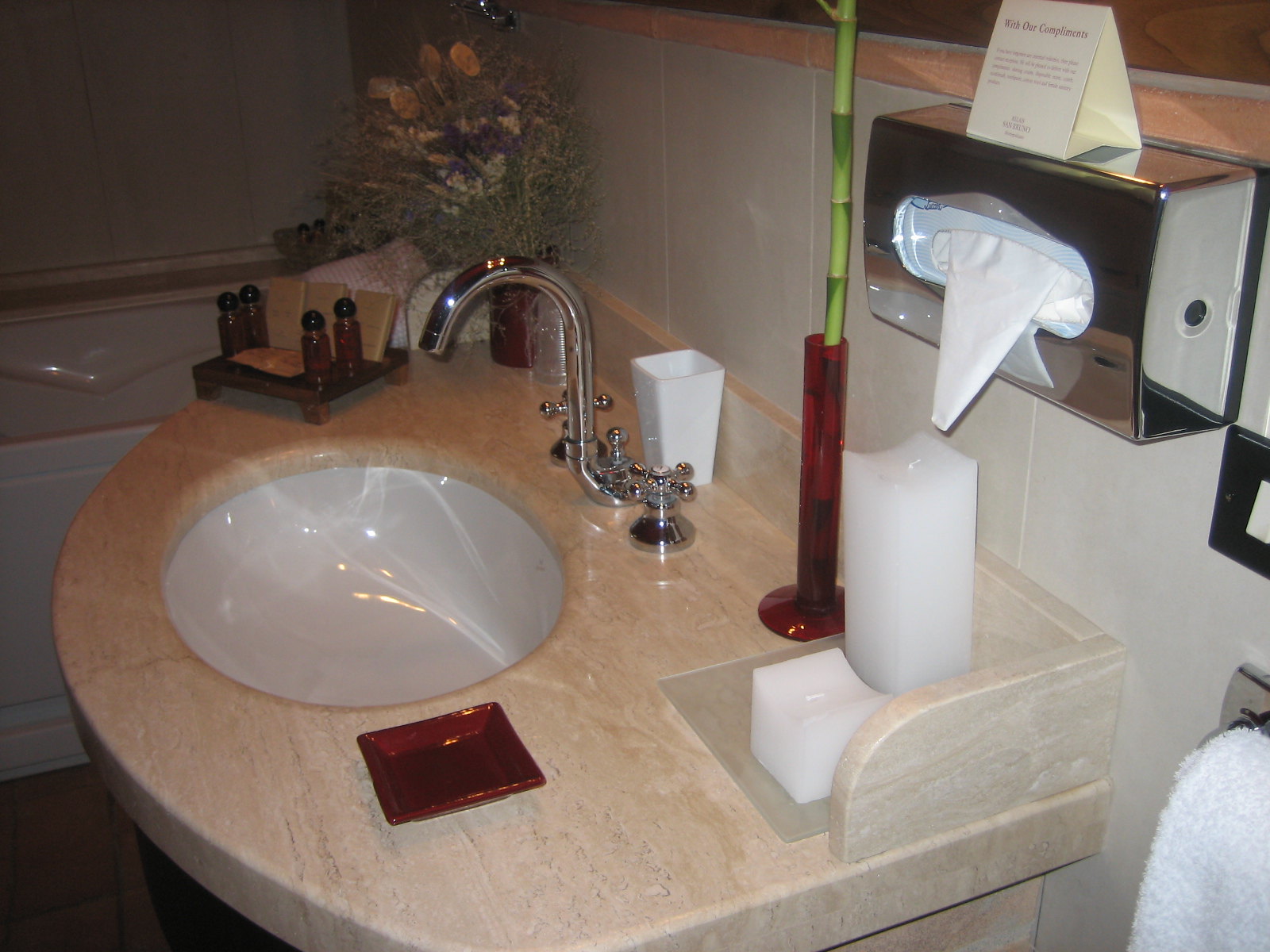The image depicts a meticulously clean bathroom, likely situated in a hotel. Dominating the scene is a pristine white vanity with sleek silver faucet and handles. On the left side of the vanity, a tasteful floral arrangement adds a touch of elegance. Partially visible to the left is the edge of a bathtub, hinting at the inviting amenities this bathroom offers. 

In front of the flowers, a tray is neatly arranged with an assortment of personal care items, including soaps, shampoos, and conditioners, ensuring guests have everything they need for a comfortable stay. Adjacent to this setup, a slender red vase containing a bamboo plant introduces a pop of color and a natural element to the room. 

Next to the vase, a white candle suggests a focus on relaxation and ambiance. Above the candle, a sophisticated silver tissue holder stands, topped with a small note that, while difficult to read, appears to offer compliments. This sophisticated arrangement further cements the impression of a well-maintained and thoughtfully appointed hotel bathroom. To the right of the tissue holder, a towel rack signifies additional convenience. The overall impression is one of immaculate cleanliness and refined comfort.